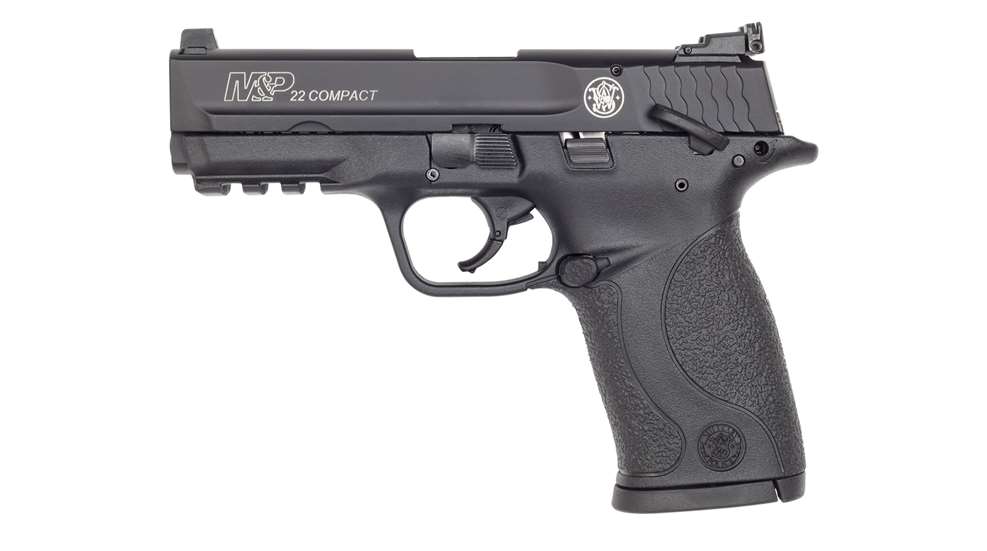The photograph displays a small, black handgun set against a stark white background, drawing attention to its detailed features. The handgun, viewed from the side with the handle on the right and the barrel on the left, is labeled "M&P 22 Compact" in white print along its side. The barrel is square-shaped and extends straight out. Notable features include the trigger positioned centrally and the different screws visible on the gun's body. There are symbols and logos on the gun, including an "M&P" inscription near the front and a small circular logo, resembling a "W," which appears on the side of the grip and near the rear of the gun. The handle's texture contrasts with the smoother barrel, highlighting the gun's compact design. The image is a clear, close-up side view that isolates the handgun against the plain background, emphasizing its real and practical design.